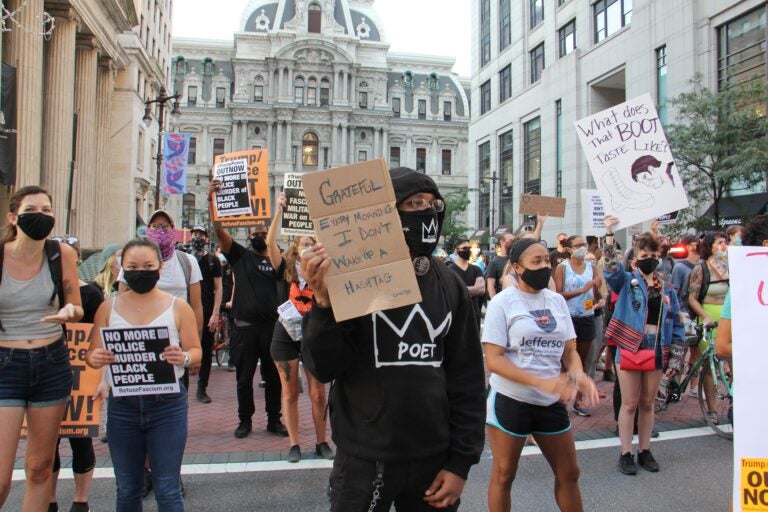This color photograph captures a vibrant Black Lives Matter march set against a bustling city block or public square. Dominating the background is a grand, ornate building reminiscent of European architecture, possibly a Parliament building. On the left side, part of a sandstone-colored structure with tall fluted columns is visible, while the right side features a more modern 1930s-style Art Deco building made of stone or concrete.

The street is densely packed with a predominantly youthful crowd, most of whom are wearing face masks due to the COVID-19 pandemic. At the forefront, a young individual dressed in a black hoodie, pants, and a black hat, all adorned with a white crown emblem, holds up a handmade cardboard sign that reads, "grateful every morning I don't wake up a hashtag." Beside them, a young woman in denim shorts and a denim top bears a sign asking, "What does that boot taste like," accompanied by an image of a boot and a man's face.

To the left, another young woman in a white tank top, blue jeans, and a black face mask displays a printed sign that protests police violence against Black people. The crowd stretches back, filled with diverse young people, many holding various signs as they march in solidarity. The image vividly encapsulates the energy and unity of the Black Lives Matter movement during a critical period in history.